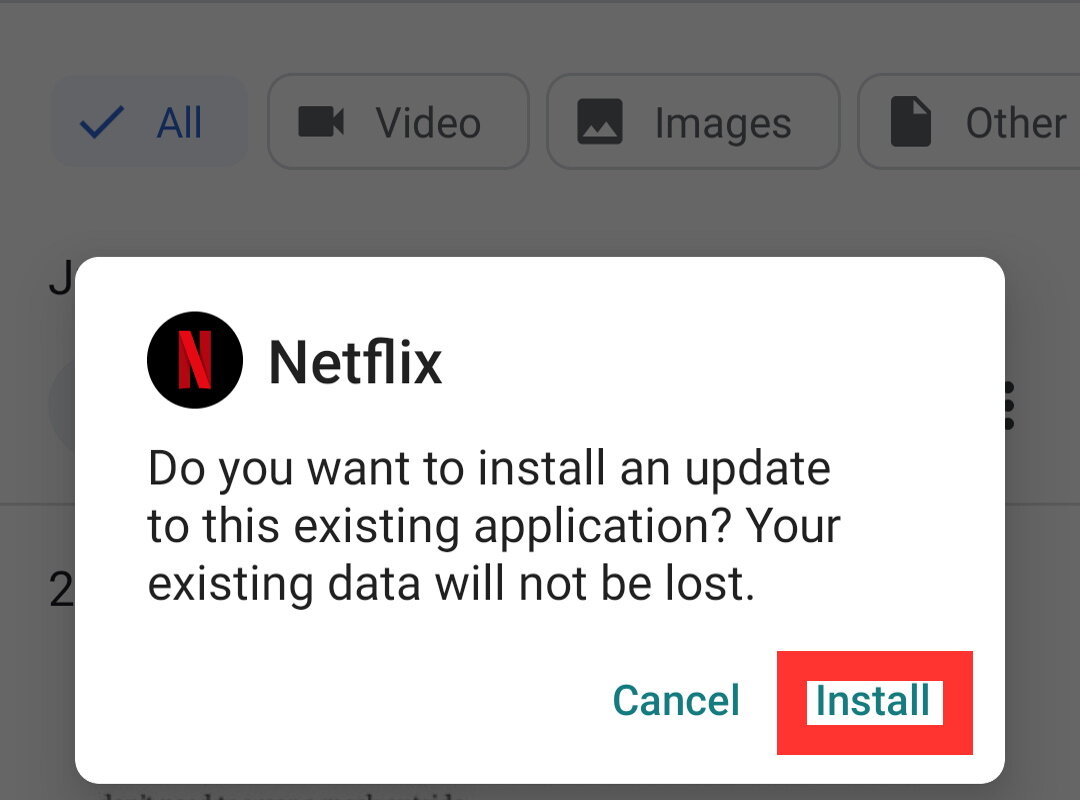The image is a rectangular screenshot, approximately 30% wider than it is tall, with the majority of the background partially obscured by a gray haze, giving a blurred effect to what appears to be a video library interface. 

At the top of the screen, a series of horizontal buttons are visible, though not completely legible. Among these buttons, the word “All” stands out in blue with a blue checkmark next to it, indicating it has been selected. 

Occupying most of the center and lower part of the image is a prominent foreground window. This window spans from about 10% from the left edge to 90% towards the right and extends from roughly one-third down the screen to nearly touching the bottom. The window has a white background and features a rectangular shape with rounded edges.

In the upper left corner of this foreground window, the newer Netflix logo is visible, consisting of a black background with a red 'N' inside a circle, reminiscent of a profile picture icon, followed by the word "Netflix." Below this logo, there are three lines of text that read: "Do you want to install an update to this existing application? Your existing data will not be lost."

In the lower right corner of the window, there are two buttons with teal text: "Cancel" and "Install." The "Install" button is highlighted with a red square around it, drawing attention as the primary action option.